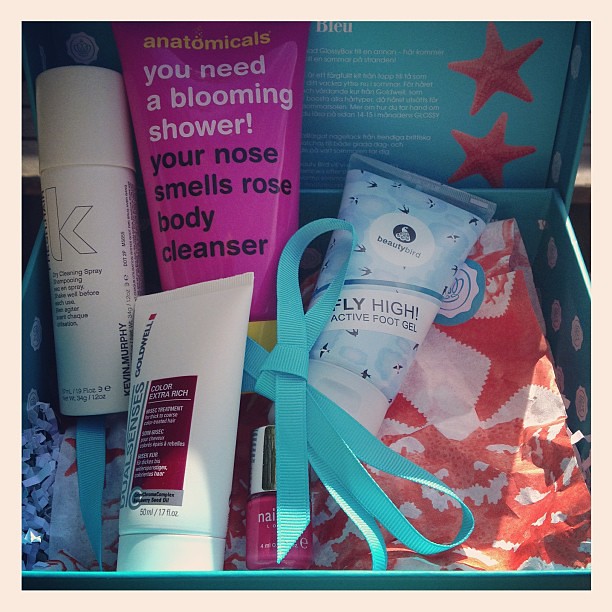The image depicts a meticulously arranged sampler box, bordered in a tannish-peach frame, accentuating its sophisticated presentation. This light blue gift box prominently features a repeated wax seal logo on the inside lid, contributing to its refined aesthetic. The contents are nestled in white crinkle paper, which serves as both packing material and additional decorative touch. Within the box are an assortment of beauty products: 

- On the left, a white canister labeled with black text and a large "K," identified as dry cleaning spray, although the brand name "Kevin Murphy" and other details remain illegible.
- To its right, a pink plastic tube from Anatomicals, bearing the playful inscription "You need a blooming shower. Your nose smells roses body cleanser."
- Below this, a white tube from Goldwell, marked "color extra rich," suggesting a product for color-treated hair.
- Tucked among them is a small tube of Beauty Bird Fly High foot gel and a pink nail polish bottle.

The scene is further complemented by a blue card with indiscernible writing, a pair of red sea stars that evoke an oceanic or nautical theme, and a scattering of white tissue paper confetti, enhancing the box’s celebratory feel. Overall, the box appears thoughtfully curated, ideal as a gift, particularly for someone with an interest in beauty and personal care products.